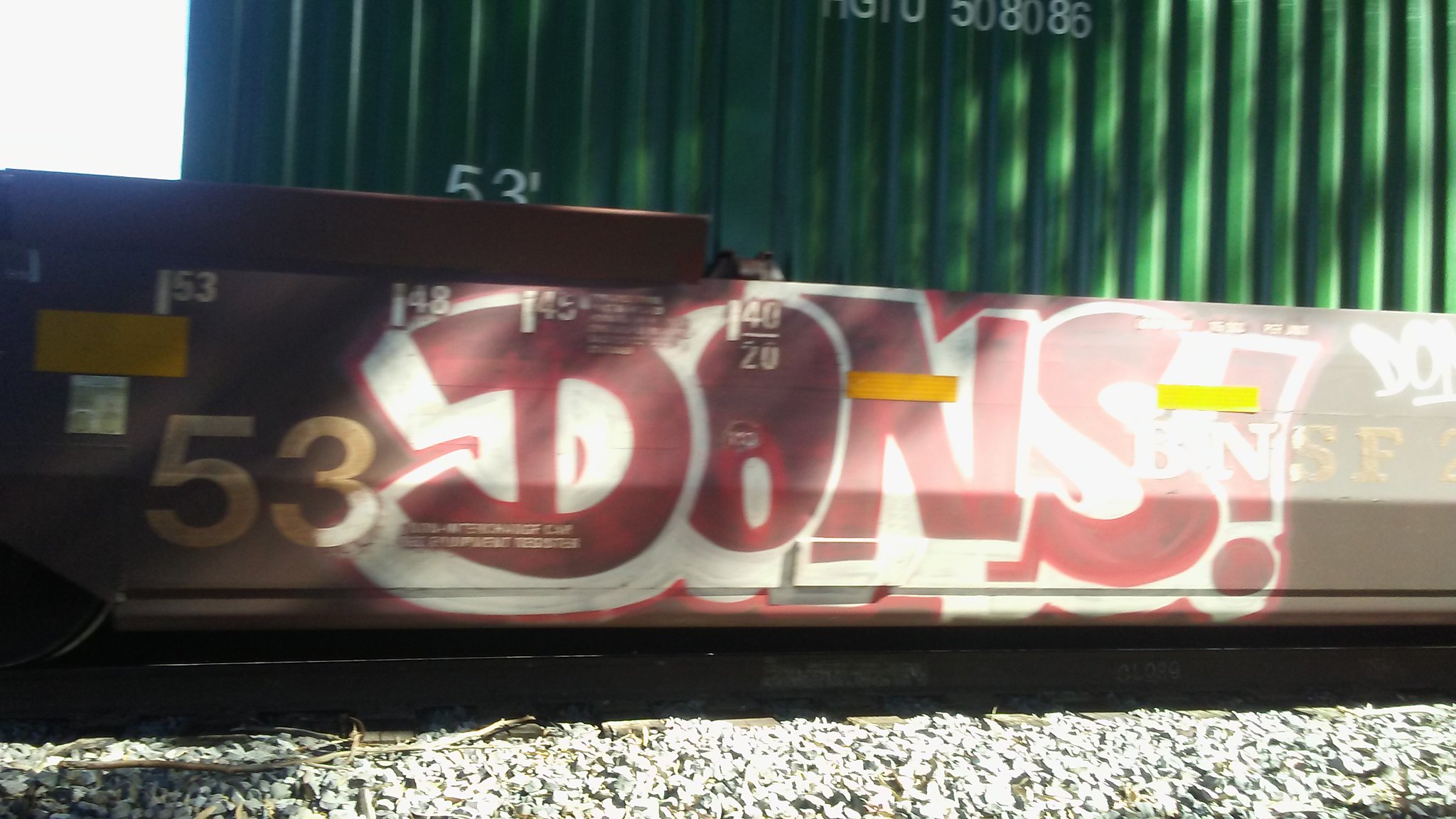This is a detailed photograph of the side of a train, focusing on a specific train car and its surroundings. The scene is set with train tracks and white stone gravel at the bottom of the image, leading up to the train car. This particular car has a brown metal body with a prominent piece of graffiti reading "DONS!" in bright red block lettering outlined in white. The lower section of the car also displays the numbers "53" alongside the initials "BNSF," which are part of the original train markings, not graffiti. Above this car, there is a green shipping container with long ridges running horizontally across it. This container is marked with the number "508086" at the top. Additionally, the background reveals a shadow that appears to be cast by a tree against the green container, adding depth to the image.